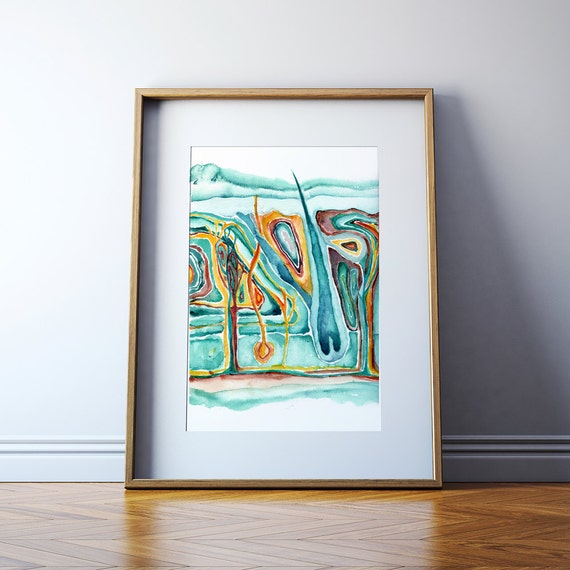This detailed painting, framed in light brown wood, exudes an abstract essence with a whirl of vibrant aqua, orange, red, yellow, green, and blue hues. Situated against a gray wall, the painting includes a white border that artfully enhances its complex interior. The painting's design evokes multiple interpretations, resembling a labyrinthine maze or a dynamic pinball machine layout. The image's intricate, swirling patterns recall cellular structures viewed microscopically: elongated and teardrop shapes, green swirls, and circular forms with blue and yellow borders. Within this abstract microcosm, elements that resemble hair follicles intersperse across a skin-like structure—albeit in unconventional colors—giving the entire piece a uniquely organic, yet surreal quality. The scene is grounded by a matching light brown wooden floor at the base of the image, harmonizing with the wooden frame of the evocative, multifaceted art piece.